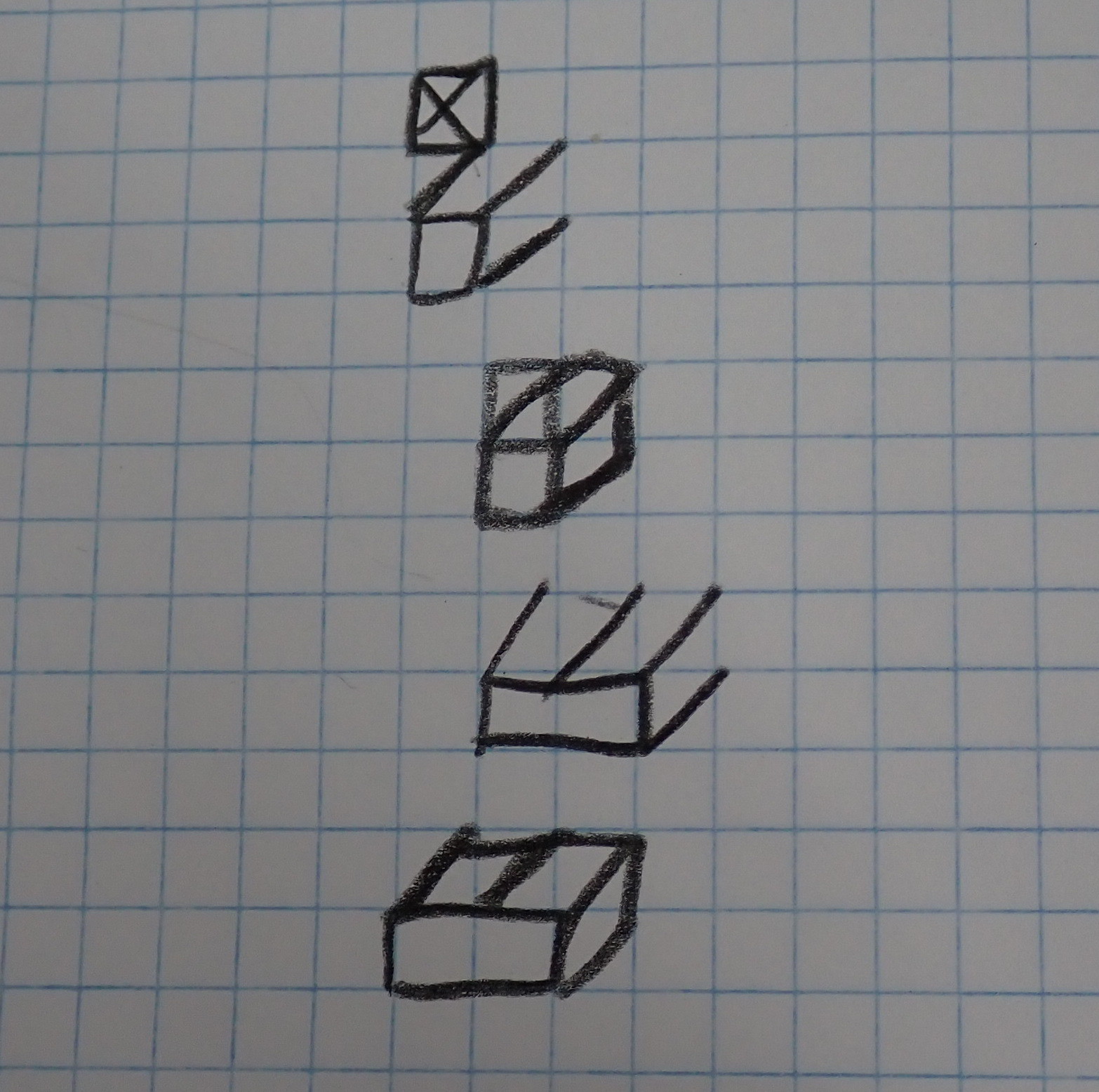This photograph features a piece of graph paper with a white background and a grid of small blue squares. At the top of the image, the second row of squares has a single square outlined in black with an "X" drawn inside it, located almost in the center of the photo. Skipping a line, the following row features another black-outlined square with a slanted line extending downwards to the line above and another line extending to the right, forming the legs of a table.

Below this, skipping another line, there are two vertically aligned squares outlined in black. To the right of these squares, slanted lines extend from the top square downwards to create legs, forming the silhouette of a table, with an additional slanted line creating a complete box structure. Lower down, skipping yet another line, two side-by-side blue squares are outlined in black. Three lines are drawn for the legs above and beside these squares.

At the bottom, there are two rows of blue squares outlined in black, resembling a cabinet with two doors. This detailed arrangement of lines and shapes on the graph paper creates various geometric designs, primarily tables and cabinets.